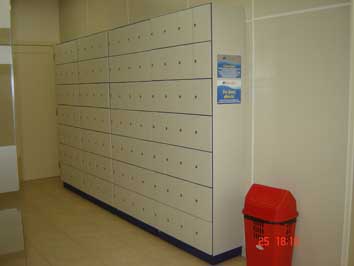This photograph, likely taken inside a building, features a beige-tiled wall with white caulk borders, creating a neutral and clinical atmosphere. On the bottom right-hand corner of the image, a red trash can with a pyramid-shaped lid draws attention; it includes a small windowed slot for disposal and sits beside a set of numbers which possibly read "2518" or "S18.18". To the left of the trash can, there is an array of small, square lockers, reminiscent of P.O. boxes or specimen boxes, typically found in medical settings. These lockers, which sport dot-patterned handles, stretch along the wall, emphasizing their uniformity and purpose. Adjacent to this bank of lockers, a poster with a gray top and a blue background, divided by a white stripe and containing some yellow possibly in the text, remains blurred and unreadable. The overall environment suggests a space designed for organization and functionality, common in institutional or medical settings.